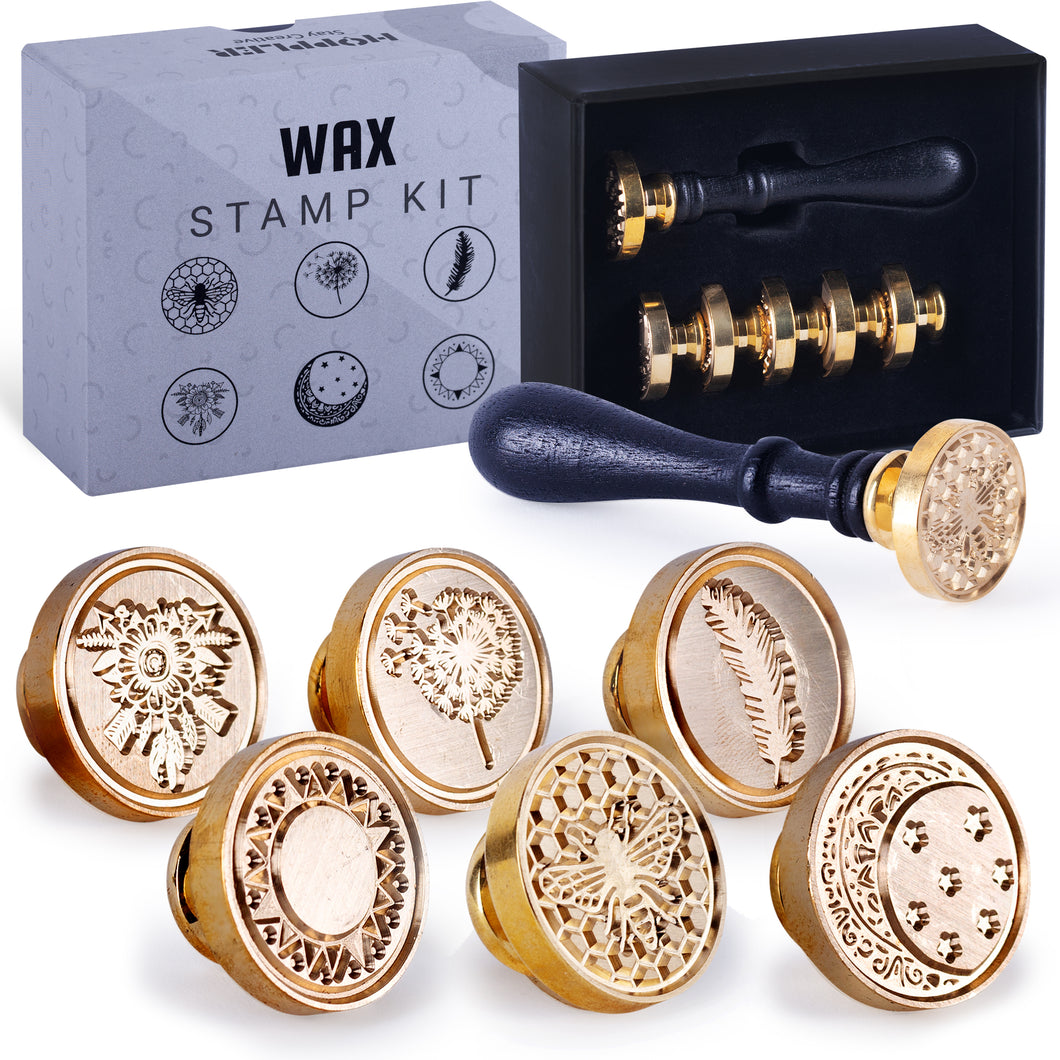This image is a detailed color photograph on a white background featuring a comprehensive wax stamp kit. On the top left of the image is the front of a light gray box with black semi-circles and bold text that reads "WAX STAMP KIT." The box showcases six circular wax stamp designs arranged in two rows of three. These designs include: a honeycomb with a bee, a dandelion with three spores blowing away, a single feather, a sunflower, a crescent moon with a lace pattern and stars, and a circle with triangular segments surrounded by dots.

To the right of this, there is an open black box revealing the complete stamp kit. The black rectangular box stands on its side, displaying the gold-topped wax stamper and the five other interchangeable gold stamp heads neatly lined up. In front of this setup, the wax stamper with one of the gold stamps attached is prominently displayed, illustrating the tool's long black handle and gold stamping head. Below all of this, a close-up section showcases the intricate details of each of the six stamp designs in larger, clearer views, emphasizing their gold finish and distinct patterns.